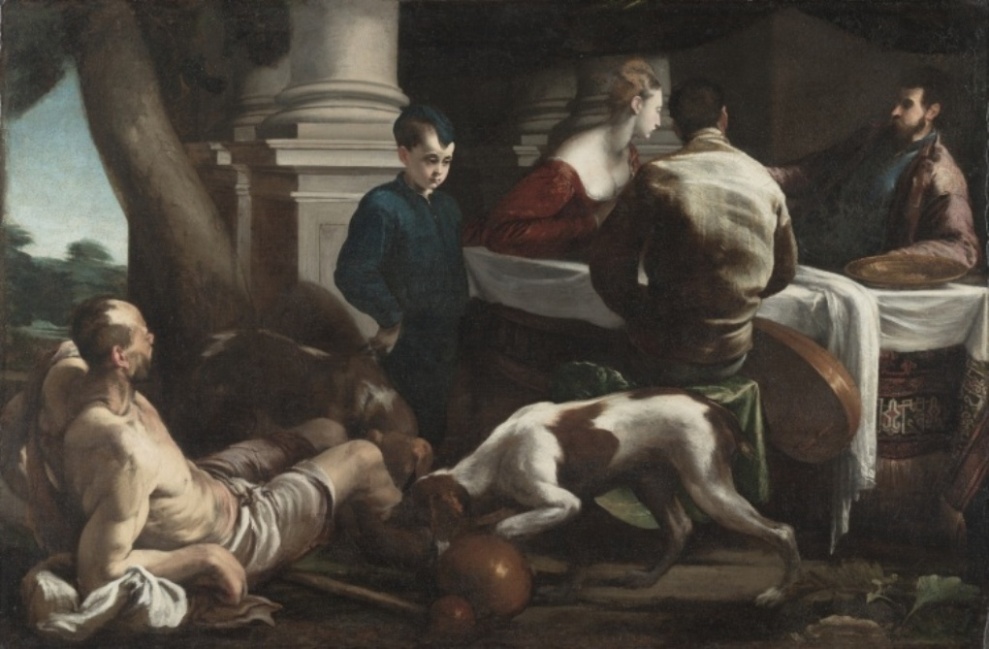This detailed oil painting, rendered in a highly realistic style, captures an indoor scene with vivid clarity. The setting appears to be a bedroom adorned with several white pillars and a glimpse of a tree branch set against a blue sky visible through a window in the background. Central to the composition is a man reclining on a bed, propped up on one arm, and partially covered by a white sheet. He wears a puffy brown jacket. Attending to him are three figures: a man seated on a green cloth-covered stool wearing a beige jacket, a boy in a dark green outfit with a matching strip of hair on his head, and a woman whose hair is swept up into an elaborate style, dressed in a striking red dress.

In the foreground, a brown and white dog with a ball captures attention. Another dog is subtly blended into the background. On the floor, another man lies mostly naked, save for a sheet draped over the lower half of his body. He is being sniffed by the aforementioned dog. Adjacent to this reclining figure stands a boy, dressed in a dark outfit, possibly blue or green, interacting with the dog.

To the right of this scene, a table with a white tablecloth is visible, around which sit three people—two men and a woman in a red dress. They appear engaged in conversation, contributing to the intimate and dynamic atmosphere of the room.